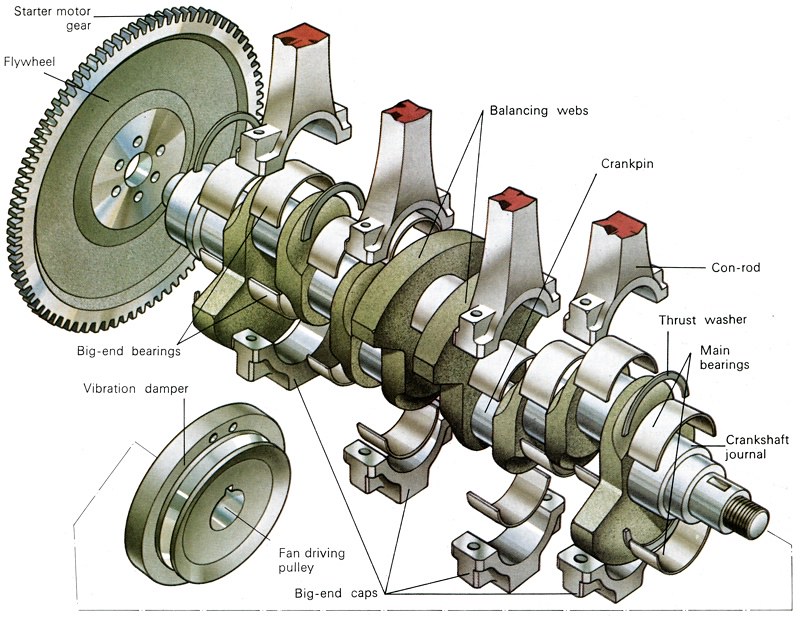The image is a detailed hand-drawn diagram showcasing the internal components of an engine. Dominating the center, the engine diagram is aligned diagonally, displaying various labeled parts integral to its mechanics. Key elements include the flywheel positioned on the far left, a large gear, mechanisms for turning the crankshaft, and other essential components such as the motor gear, balancing webs, crank pin, conrod, thrust washer, main bearings, crankshaft journal, big end bearings, vibration damper, fan driving pulley, and big end caps. The diagram is meticulously detailed, with the colors black, white, gray, tan, brown, silver, and a reddish hue contributing to the illustration’s clarity and depth.